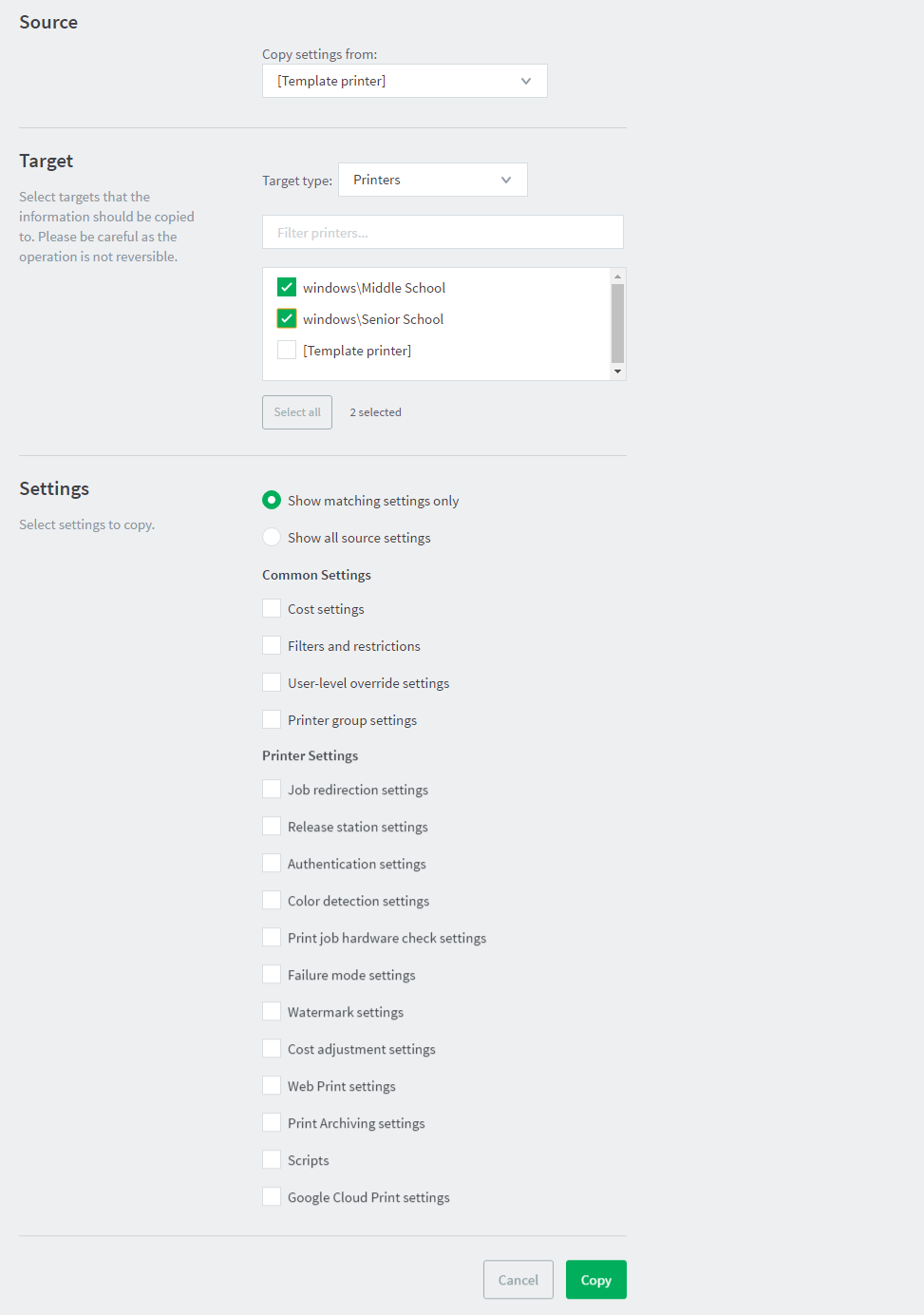Sure! Here's a cleaned-up, detailed caption:

---

Screenshot of a Source Settings Page for Printer Configuration

This image captures a screenshot from a printer configuration source page with a light gray background. In the upper left corner, the word "Source" is displayed in black text. Centered at the top is the label "Copy Settings From," followed by a rectangular drop-down menu labeled "Template Printer."

Below this, on the left side of the screen, black text instructs users to "Select targets that the information should be copied to. Please be careful as the operation is not reversible." To the right, there is another label reading "Target Type," paired with a drop-down menu set to "Printers."

Beneath these instructions lies a rectangular filter labeled "Filter Printers." Directly below the filter is a list contained within a rectangular window, showing entries such as "Windows Middle School," "Windows Senior School," and "Template Printer."

Further down, two buttons labeled "Select All" and "To Selected" can be found. On the lower left side is the "Settings" section, prompting users to "Select settings to copy." To the right, several categories are listed: "Show Matching Settings Only," "Show All Source Settings," "Common Settings," "Cost Settings," "Filters and Restrictions," "User Level Override Settings," "Printer Group Settings," "Printer Settings," "Job Redirection Settings," "Release Station Settings," "Authentication Settings," "Color Detection Settings," "Print Job Hardware Check Settings," "Failure Mode Settings," "Watermark Settings," "Cost Adjustment Settings," "Web Print Settings," "Print Archiving Settings," "Scripts," and "Google Cloud Print Settings."

At the very bottom of the screenshot, there are two buttons labeled "Cancel" and "Copy."

---